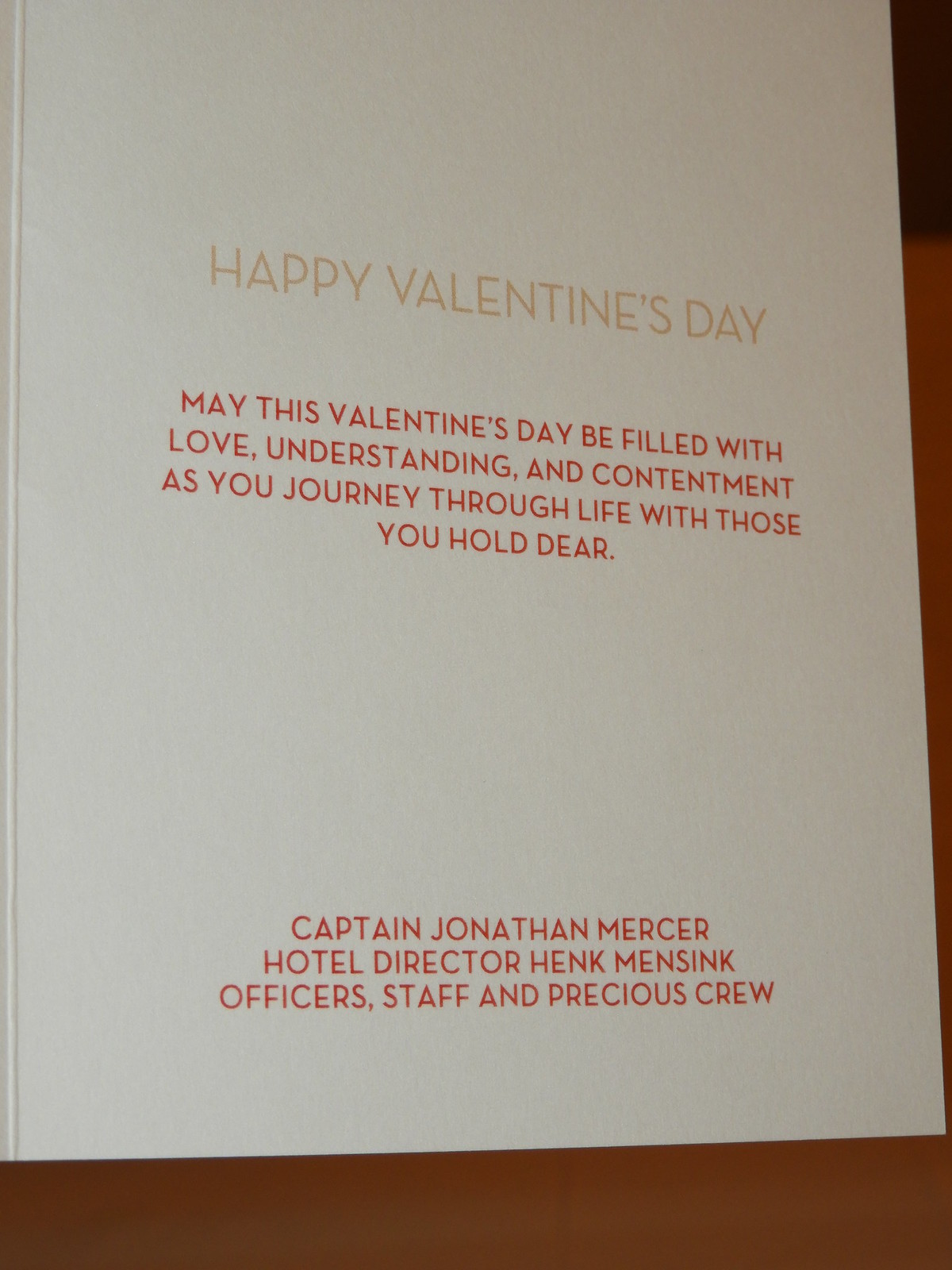The image depicts a color photograph of the inside of a vertically aligned Valentine's Day card resting on a dark brown wooden table. The card, which is white and has ample blank space, features an inscription in a brownish-gold font at the top that says, "HAPPY VALENTINE'S DAY." Below this, in red text, it reads: "May this Valentine's Day be filled with love, understanding, and contentment as you journey through life with those you hold dear." At the bottom of the card, also in red font, it lists "Captain Jonathan Mercer," followed by "Hotel Director Hank Mensink," and then "Officers, Staff, and Precious Crew." The card is slightly angled to the top left, and the detailed, centered text is arranged to convey a heartfelt message. The background surface where the card rests is solid black at the very bottom, adding contrast to the overall composition.